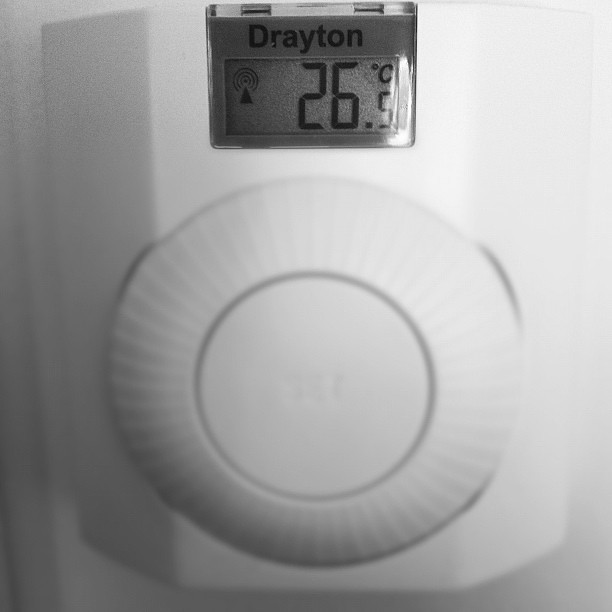This image features a detailed close-up of a white, square-shaped digital thermostat. Prominently displayed in the center is a circular dial with line indicators, suggesting an adjustable setting that likely rotates to control the temperature. The upper portion of the thermostat is gray, bearing the brand name "Dryton" in black text. Just below the brand name, the current temperature reads "26.5°C", with the ".5" in smaller font. To the right of the temperature display, there is a black triangle icon, encircled by three lines that presumably indicate wireless signal strength or connectivity. A small black dot is centered within the upper part of the triangle design. Additionally, there is a noticeable shadow cast along the left side of the device, adding depth to the image.